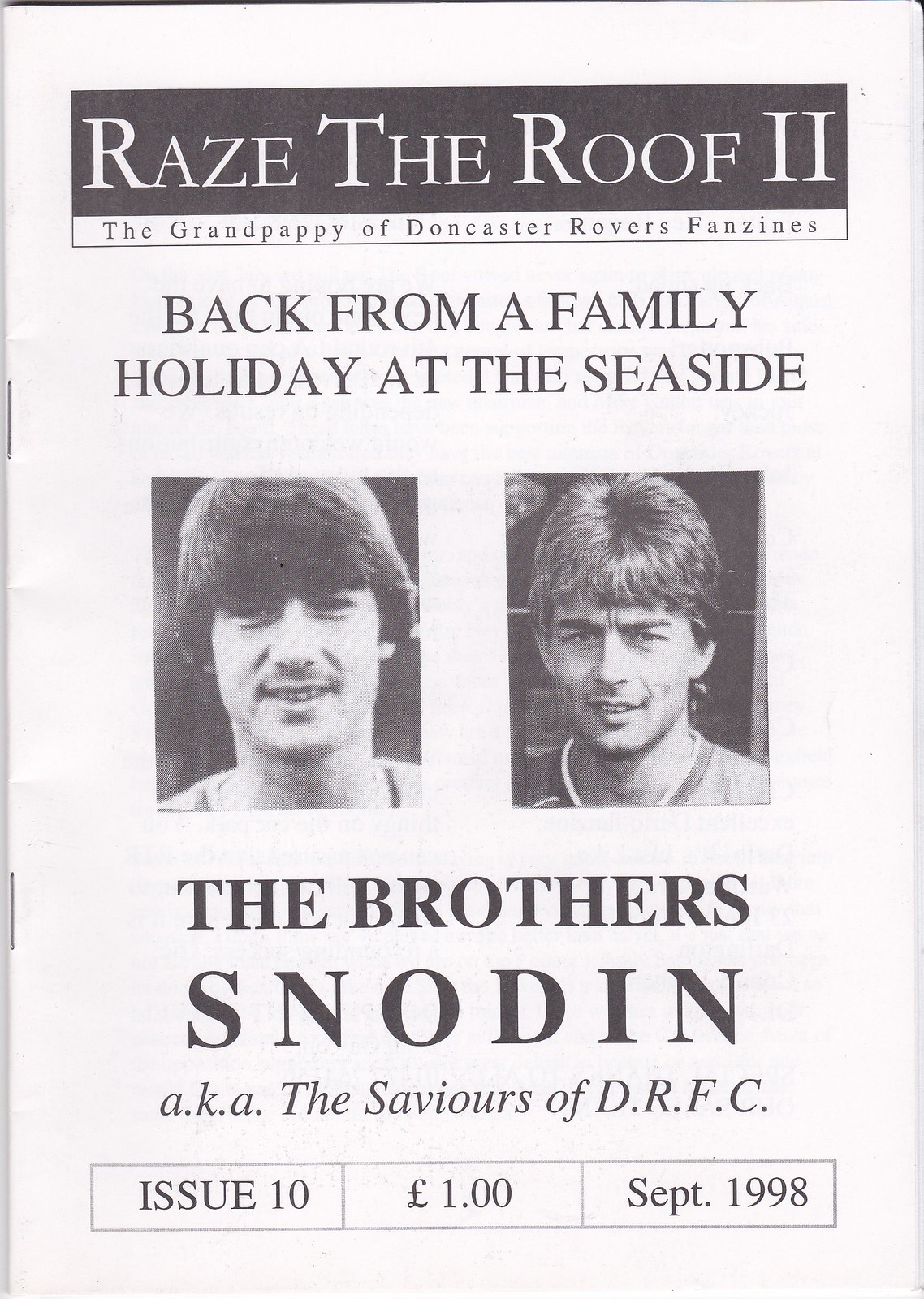This is a black-and-white vertical rectangular cover, likely of a magazine or program, featuring a prominent black banner across the top with white letters that read "Raise the Roof II," with "Raise" spelled "R-A-Z-E." Below that banner, in smaller print, it reads "The Grand Pappy of Doncaster Rovers Fanzines." The cover predominantly shows a black-and-white photo of two men, identified as "The Brothers Snowden," who seem to be players of the Doncaster Rovers Football Club. A caption below the photo states "Back from the Family Holiday at the Seaside," and also refers to the brothers as "The Survivors of D.R.F.C." Additional details at the bottom of the cover indicate that this is Issue 10, priced at £1, and was published in September 1998.